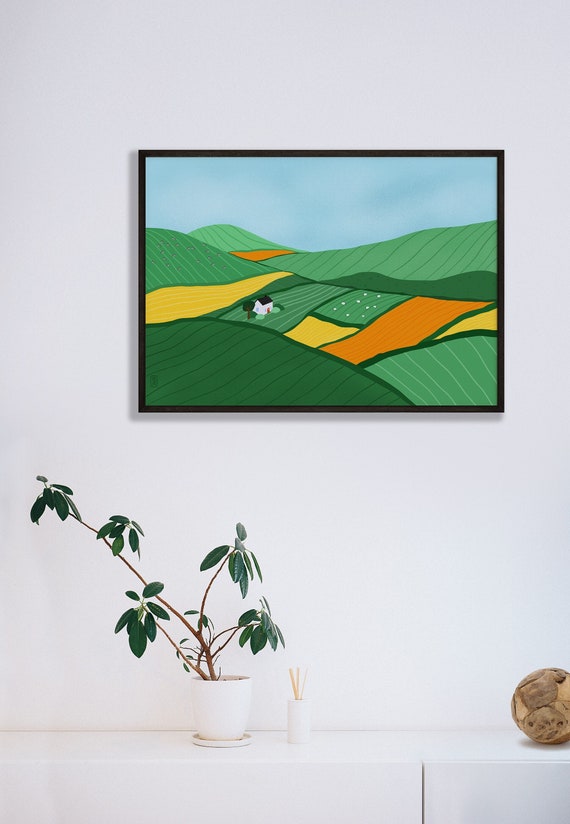This image depicts a section of a living room centered around a white wall adorned with a detailed painting of a farming landscape. The painting showcases rolling green hills, a small white house with a red door and black roof, and geometric yellow and orange fields under a blue sky. The colors in the artwork are vivid yet simple, with no shading. Beneath the painting, on a ledge or countertop likely part of a TV stand, sits a small white potted plant with green leaves. To the right of the plant, there is an oil-infused air freshener and a brown leathery ball with a patchwork texture resembling wooden bark. This arrangement underscores a cozy and stylish domestic setting.